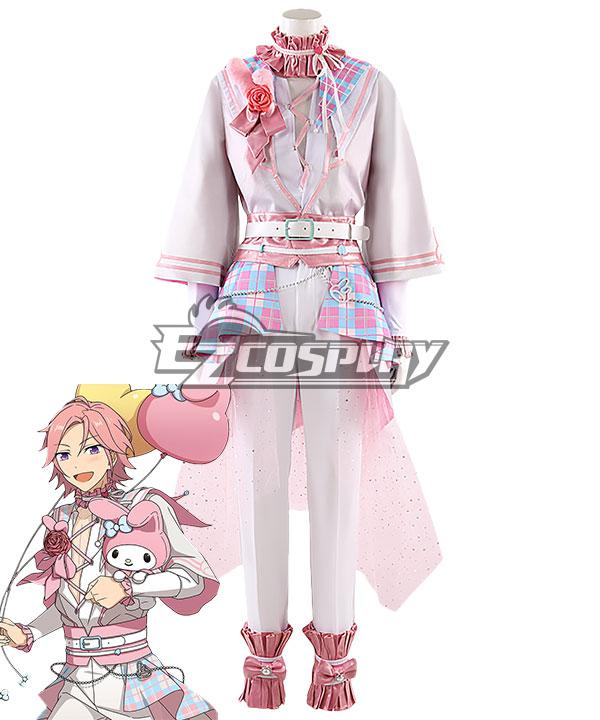This advertisement showcases a meticulously designed anime-inspired costume set on a white, headless mannequin against a white backdrop. The outfit prominently features a light lavender half-kimono jacket adorned with dark pink stripes on the lapel and cuffs, and is fastened with a white belt. Embellishments include a pink ribbon, a rose, and a dark pink neck kerchief. The skirt contrasts strikingly with its plaid pattern in light blue and dark pink tones. Completing the ensemble are dark pink leg warmers. Further detailing includes a sheer, sparkly tail-like extension from the kimono, and a chain accessory. Accompanying the display is a cartoon depiction of the character in the same outfit, emphasizing the costume's source material. The lower right corner features a watermark reading "EZ Cosplay," reinforcing the brand association. This feminine, detailed costume is designed to bring an anime character to life, making it an ideal choice for cosplay enthusiasts.